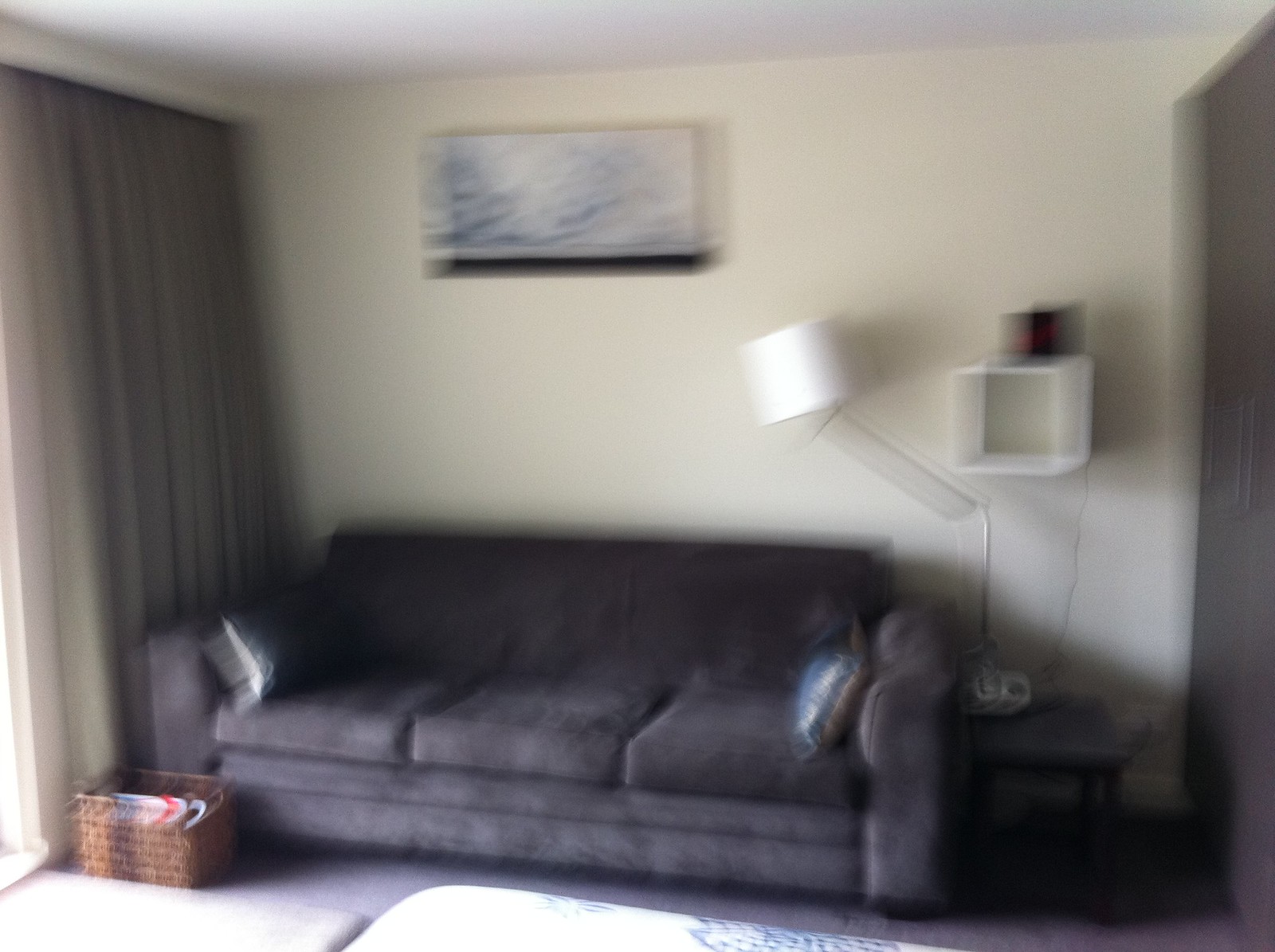The photograph depicts a slightly blurry view of a cozy living room. The walls are painted in a warm beige tone, setting a calming backdrop for the room's furnishings. The centerpiece is a gray sofa, adorned with two throw pillows for added comfort. To the left of the sofa is a brown wicker basket, though its contents remain indistinguishable. 

Above the sofa, a piece of art is mounted on the wall; its details aren't clear, adding an element of mystery to the space. To the right of the artwork, a wooden cube is affixed to the wall, serving as a functional storage solution. Atop this cube is an unidentifiable dark object. 

The right side of the image reveals a darker area, where a doorway can be seen, suggesting an entrance to another room. A slanted, slightly crooked lamp extends over the couch, providing ambient lighting. On the far left, a set of French doors, or a large window dressed with dark green curtains, adds depth and dimension to the room.